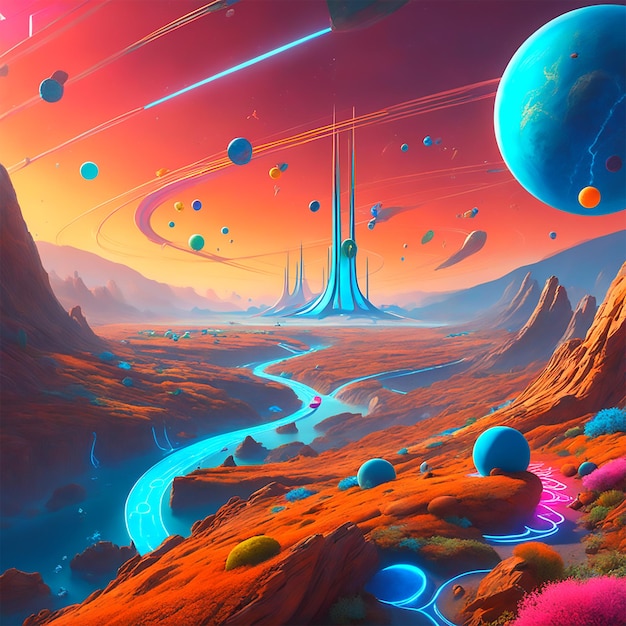This image depicts a vividly colorful, computer-generated scene of a fantastical alien landscape, possibly created using AI. Dominated by a futuristic vibe, the scene is awash with neon hues of orange, blue, and pink. The main feature is a vast, reddish-orange planetary surface, accented by luminescent vegetation, notably pink bushes. Central to the composition is a fluorescent blue river that winds its way from the foreground to a striking tower-laden city in the middle ground. These towers, resembling sharp needles or spires, suggest a complex architectural structure that might be part of an alien metropolis.

The sky is a dazzling spectacle, displaying a vibrant palette of red, orange, and yellow. A prominent blue planet hovers in the upper right corner, its size and color making it a focal point amidst a scattering of smaller, multicolored planetary bodies. Additionally, thin, orbit-like stripes wrap around the sky, adding to the otherworldly ambiance. The ground is bordered by mountains, creating a natural frame that further emphasizes the depth and surreal quality of this extraterrestrial environment.